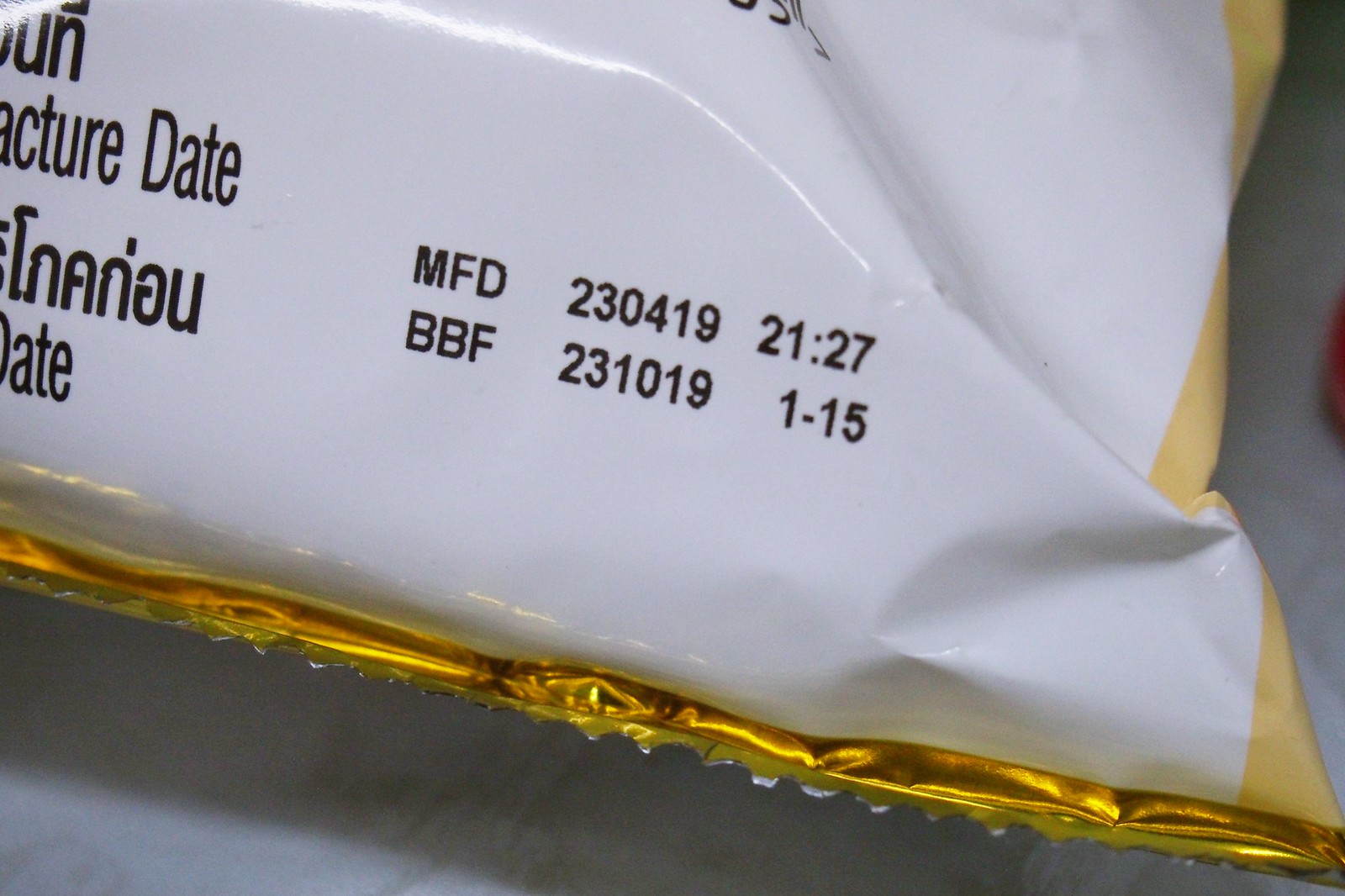The photograph captures a close-up view of the lower right corner of a bag, likely containing chips or snacks. The front of the bag is predominantly yellow, trimmed with a gold lining along the bottom edge. The back of the bag is white, featuring black text indicating key dates. In the bottom right corner, the text reads "MFD 230419 2127" and "BBF 231019 1-15", which denotes the manufacturing date of April 23, 2019, at 21:27, and a best before date of October 19, 2023. Additionally, there are some letters, possibly in Thai or Vietnamese, alongside English labels such as "manufacture date" positioned on the left side of the corner. The bag appears to be placed on a white table, and a small part of a person's finger is visible near the edge of the image.